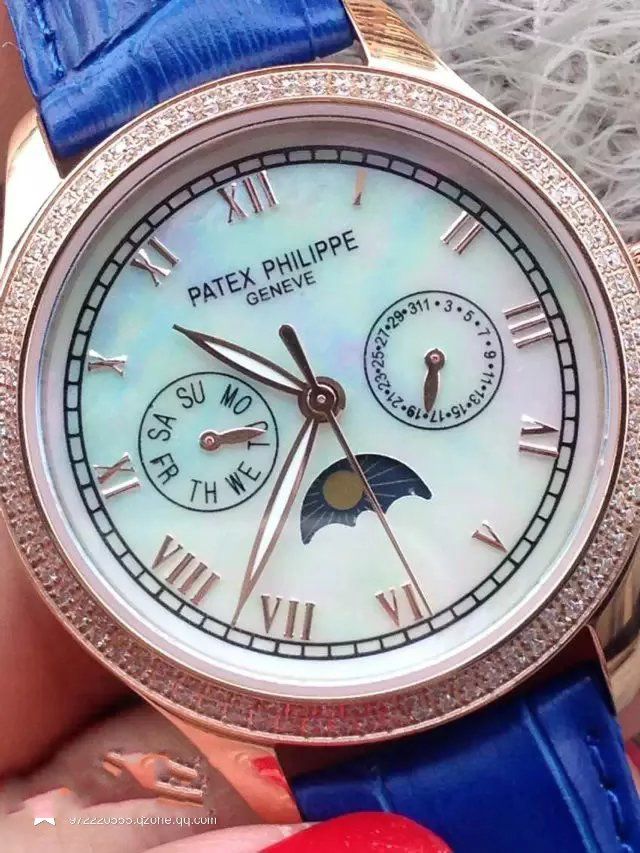The image depicts a watch face with a sleek, elegant design. The main dial is white and features abbreviated days of the week: "S", "A", "S", "U", "Mo", "Tu", "We", "Th", and "Fr," presumably standing for Saturday, Sunday, Monday, Tuesday, Wednesday, Thursday, and Friday. 

At the bottom of the watch face, there is a celestial logo representing the phases of the moon or the sun's position, indicating the time of day. On the right side of the dial, there is a date meter that displays the numbers 1 through 31, helping track the day of the month. 

At the top of the watch face, the brand "Patek Philippe" and the name "Geneva" are inscribed, signifying an association with the renowned Swiss watchmaker. The watch band is made of blue leather, enhancing its sophisticated aesthetic. The outer edge of the watch features a rose gold finish, providing a luxurious contrast to the white background of the watch face.